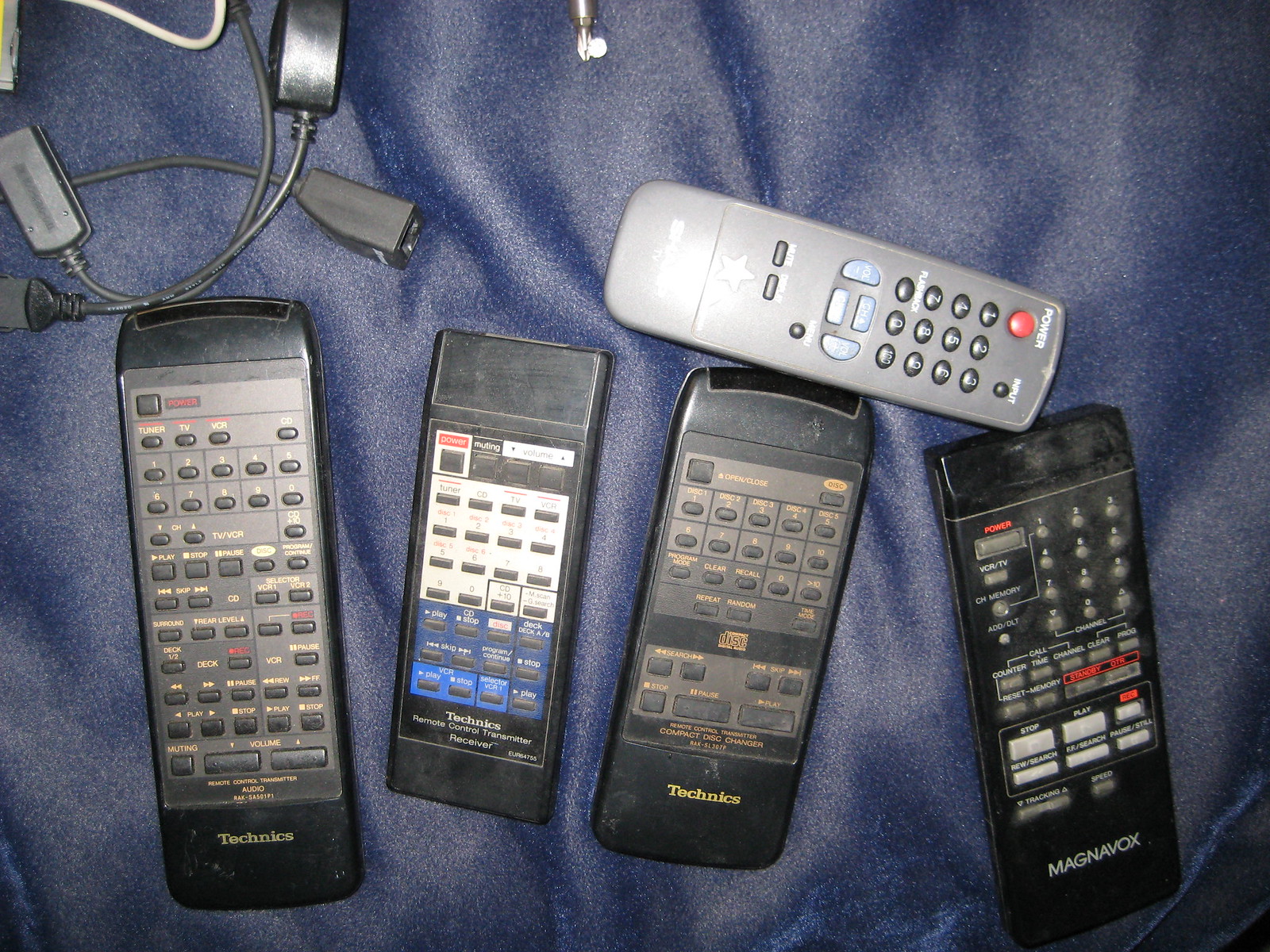This photograph presents a collection of five vintage remote controllers, predominantly black, laid out on a rippled blue fabric background, possibly a blanket or tablecloth. Four of the remotes are aligned vertically and nearly parallel to each other, while a fifth, smaller, silvery-gray remote (an old cordless phone with black and red buttons) rests horizontally atop the rightmost two remotes, acting as a visual focal point. The remotes appear to be brands like Technics and Magnavox, indicative of mid-1980s to early 1990s technology. The blue fabric beneath them is slightly wrinkled, adding a textured background to the scene. In the upper left corner, there are assorted audio-visual cables and adapters potentially related to the remotes or phone, and the tip of a Phillips head screwdriver protrudes into the frame from the top center, suggesting a workspace or a repair environment. The remotes themselves appear well-used and somewhat dirty, adding to the nostalgic and vintage feel of the image.